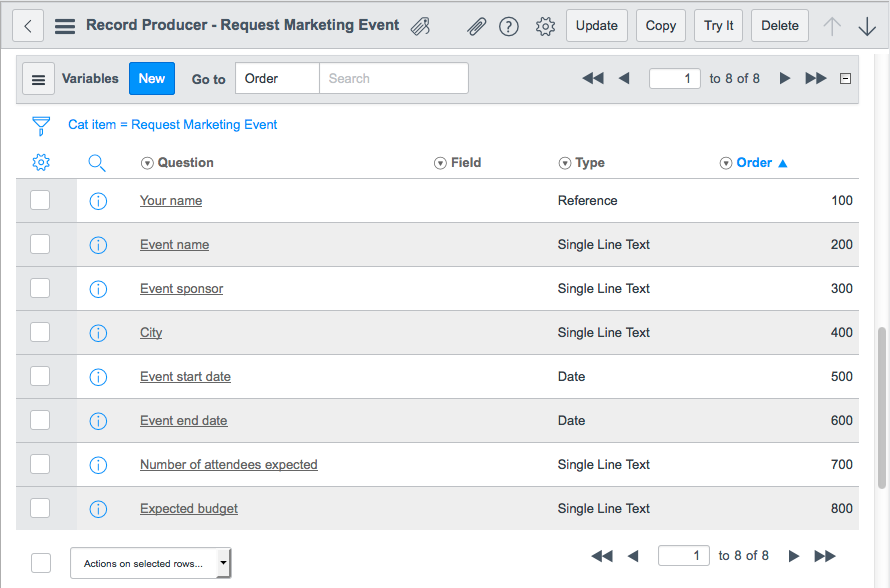The screen capture depicts a user interface of a website designed for managing marketing events. The browser window frame is grey, while the central area has a clean white background. Dominating the top portion is a grey banner that reads "Record Producer Request Marketing Event." To the right of this title, there are several icons including a sales tag, a circle with a question mark, a settings gear, and four grey horizontal buttons labeled "Update," "Copy," "Try It," and "Delete" in black text. Adjacent to these buttons is a highlighted grey down arrow.

Beneath the primary banner, a secondary grey line features labels such as "Variables," "New," and "Go To," with "New" residing inside a blue square with white lettering. Next to the "Go To" label, there is a white bar displaying the word "Order" in bold black text on the left, and the word "Search" on the right. On the right-hand side of this bar, navigation arrows for moving back and forward flank a small white box marked with "1" and the text "128 of 8."

In the white main section, starting at the top left corner in blue text, it says "Cat Item Equal Request Marketing Event." Below a blue settings gear icon on the left is a grey column containing empty white checkboxes. Across the top right section, the interface includes a blue search glass icon followed by labels: "Question" in black, "Field" in black, "Type" in black, and "Order" in blue. The rows listed below this header alternate in color between white and grey, and are populated with various questions such as "Event Start Date," "Event End Date," and "Number of Attendees Expected." Under the "Type" column, it indicates data types such as "single line text" and "date." In the "Order" column, the sequence starts at 100 and increments by 100 with each row until reaching 800.

At the bottom of the screen, the navigation area with back and forward arrows and the "128 of 8" text is repeated. In the bottom left corner, on a white background, there is a drop-down box labeled "Actions on Selected Rows." This detailed layout facilitates detailed management and tracking of marketing event requests.